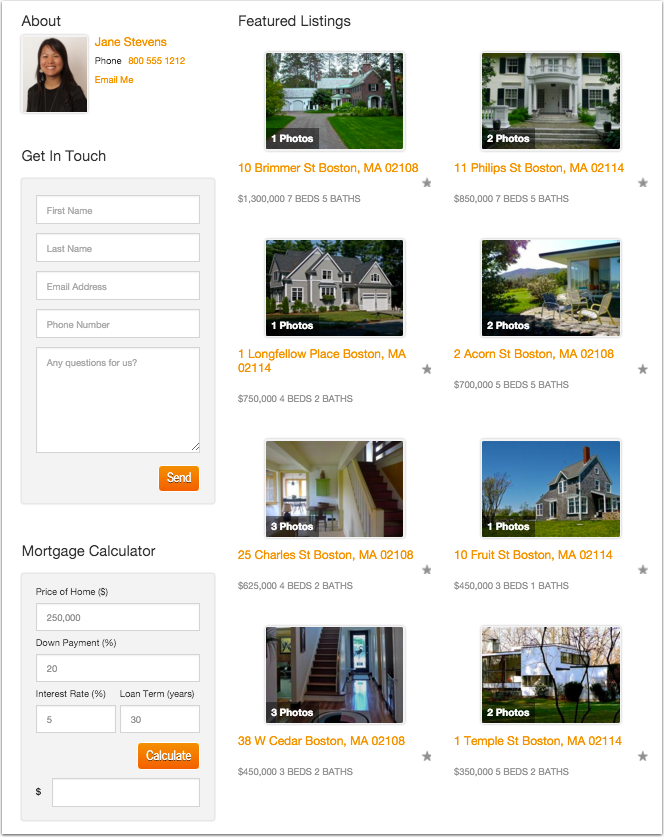**Screenshot of Realtor Jan Stevens' Personal Realty Website**

This screenshot captures a detailed view of realtor Jan Stevens' personal page on a realty website. The page prominently features eight listings, all located in Boston, Massachusetts, with properties ranging in price from $350,000 to $1.3 million.

On the left side of the page is a comprehensive "About" section. This section includes a professional profile picture of Jan Stevens, a young female realtor. Her contact information is also displayed, including her phone number and an email link. Below her profile picture, there is a contact form where visitors can enter their name, email, phone number, and a short message to get in touch with her.

Additionally, beneath the contact form, there is a mortgage calculator tool. This tool allows potential buyers to estimate their mortgage payment by inputting the purchase price, down payment, interest rate, and loan term.

The eight featured listings are presented prominently, showcasing a diverse range of properties suited for various budgets and preferences.